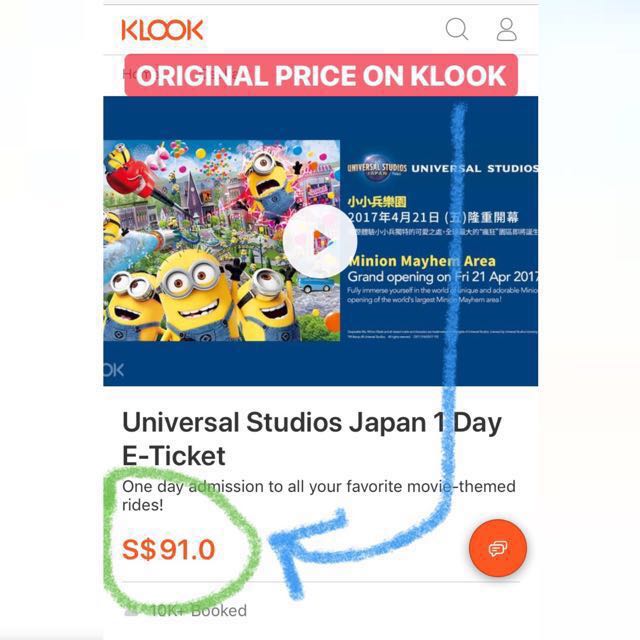This image is a detailed screenshot of the KLOOK website, featuring a promotional section for Universal Studios Japan. The top white navigation bar prominently displays "KLOOK" in red capital letters. Beside it on the right are a magnifying glass and a profile icon. Below the top bar, there is a red banner with white bold capital letters stating "ORIGINAL PRICE ON KLOOK."

Beneath the banner is a dark blue box. On the left side of this box is an image from the "Minion Mayhem" area of Universal Studios Japan, featuring a collage from the Despicable Me movies. Overlaid on this image is a white circular play button icon. To the right of the image, the Universal Studios logo is displayed alongside the text "Universal Studios" in white, bold capital letters.

Below the Universal Studios logo, there's text in yellow Chinese characters, followed by "2017" next to several other Chinese characters, including numbers "21" and characters in parentheses. Further down, in small white Chinese text, there is a string of characters that are hard to read due to the size. Below this, in bold yellow text, it reads "Minion Mayhem Area." Underneath it, white text states, "Grand Opening on Friday, 21 April 2017."

A descriptive text in smaller white italic font follows: "Fully immerse yourself in the world of the works' unique and adorable Minions with the opening of the world's largest Minion Mayhem area." Underneath, smaller pixelated text is illegible.

To the bottom left, parts of light blue letters "O" and "K" are visible, partially cut off, over a dark blue background. Below the dark blue box, bold black text announces "Universal Studios Japan One Day E-ticket," with a subtext in regular black text saying "One-day admission to all your favorite movie-themed rides." Below this is a price listed in red text "$91.0," circled in green crayon.

An arrow drawn in blue crayon points from the top of the dark blue box straight down to the circled price. On the right side, a red circle with conversation box icons appears, and a gray line extends across the bottom with the text "10K+ BOOKED."